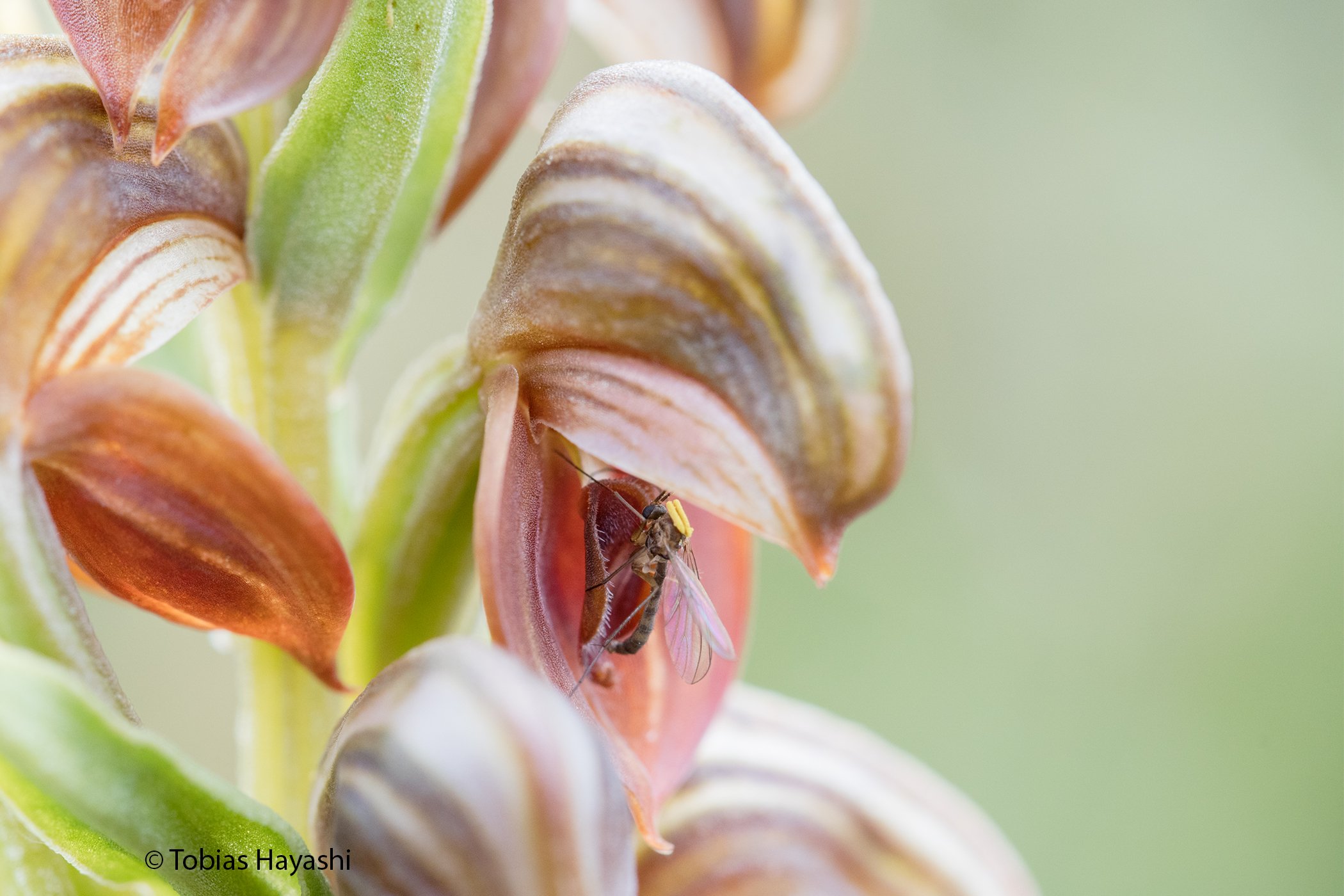The image is a highly detailed, close-up photograph of an insect nestled within a unique flower. On the left-hand side, green plant stems dominate the scene, adorned with moon-shaped flowers. These flowers have a distinctive appearance: their tops are brownish, while the petals underneath carry a bacon-like hue. Among these flowers, there's a particular one featuring the focal point of the image – an insect that looks somewhat like a wasp but could also be a bee. This insect has a slender, brownish body and clear wings, and it seems to be either trapped or resting within the flower. The depth of field in the photograph is very pronounced, rendering the background into a soft, blurry field of olive green, accentuating the intricate details of the plant and insect on the left.